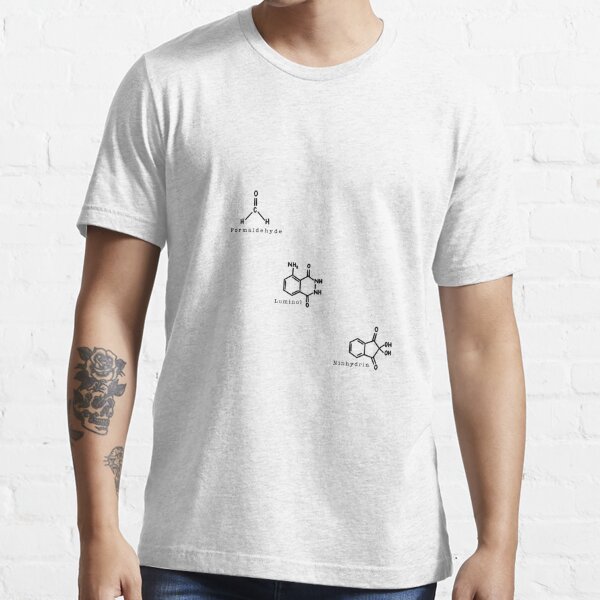The color photograph, in portrait orientation, features a male model modeling a white crew-neck t-shirt with short sleeves. The model is pictured from the neck down to about mid-hip, standing against a white brick wall. The t-shirt displays three chemical symbols arranged diagonally across the mid-chest area. Each symbol is outlined in black with small, illegible text underneath. The man's left forearm sports a tattoo of a skull and a rose, while his inner arm, closer to the wrist, bears another indistinguishable tattoo. The model is also wearing blue jeans. The overall style of the image falls under color photographic representationalism, realism, fashion photography, and product photography.